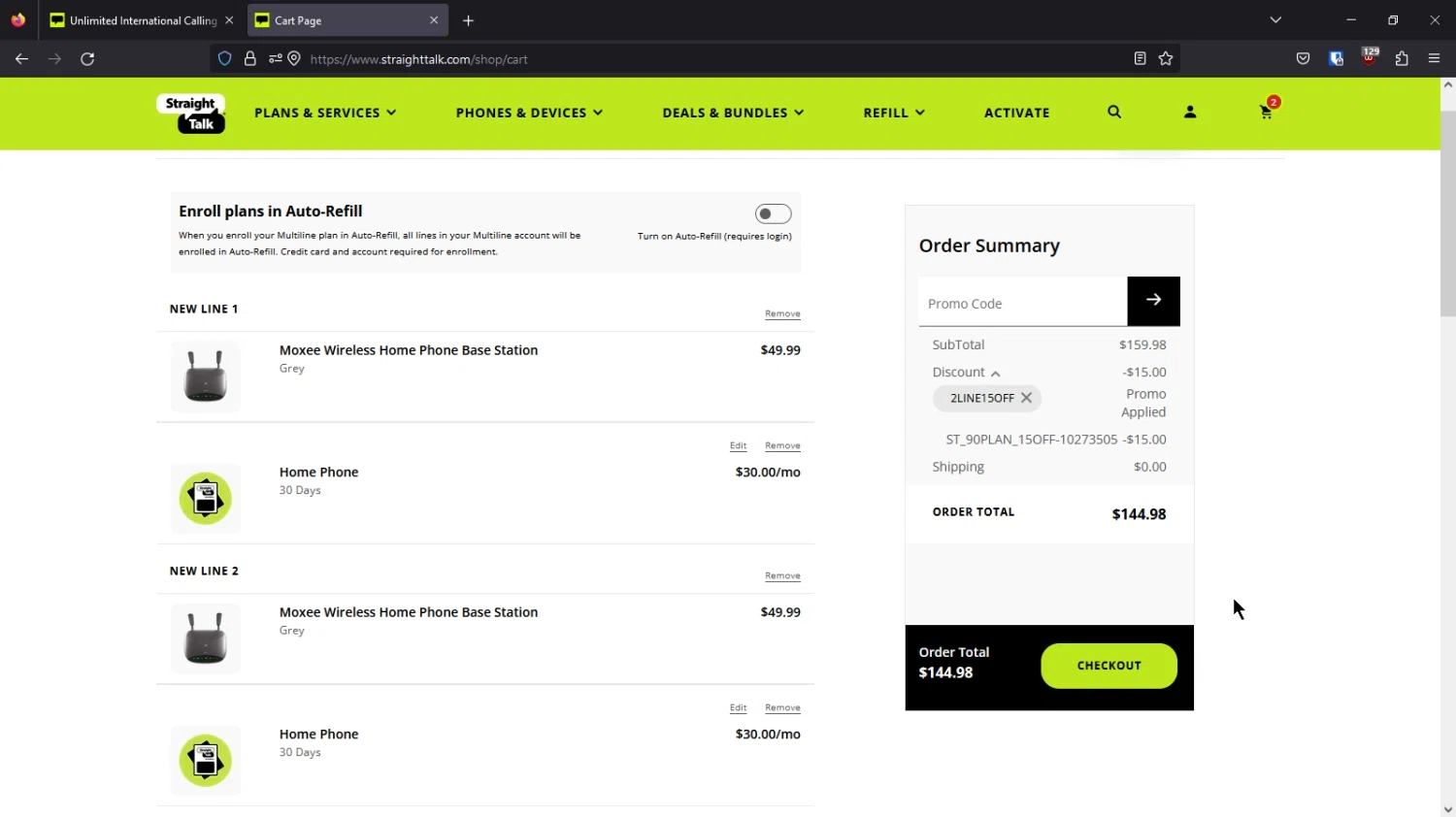This image is a detailed screenshot from a website, specifically Straight Talk's shopping cart page, viewed using the Firefox browser. At the top, within a black navigation bar, two browser tabs are open: "Unlimited International Calling" (currently active) and "CART page." The familiar Firefox emblem is visible on the far left. 

Directly below, the address bar displays the URL: straighttalk.com/shop/CART. Beneath it is a prominent lime green navigation bar, adorned with the Straight Talk black and white logo on the left. Adjacent to the logo, a series of black text pull-down menus offer categories such as "Plans and Services," "Phones and Devices," "Deals and Bundles," "Refill," and "Activate."

A section explaining enrollment plans and auto-refill follows: "Enroll Plans and Auto-Refill. When you enroll your multi-line plan and auto-refill, all lines in your multi-line account will be enrolled in auto-refill. Credit card and account required for enrollment." Notably, the auto-refill option is toggled off.

Below this, the product details are listed in a semi-structured format:

- **New Line 1:** Moxie Wireless Home Phone Base Station (gray). **Price:** $49.99. Accompanying it is an image of the device, featuring two antennas. **Plan:** Home Phone for 30 days. **Price:** $30/month.
- **New Line 2:** Identical to New Line 1 with the same device and pricing.

On the right-hand side, an "Order Summary" section provides an overview:
- **Subtotal:** $159.98
- **Discount:** -$15 (promo code applied: Line 15 off)
- **Shipping:** $0
- **Total:** $144.98

A green "Checkout" button is prominently displayed at the bottom of this section.